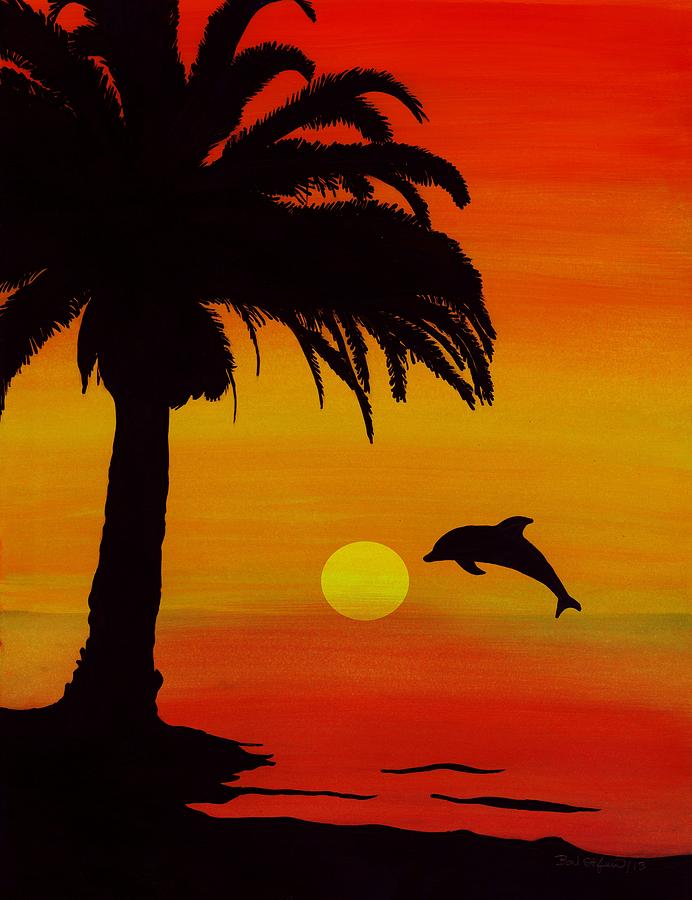This vibrant painting, likely done in oil or acrylic, captures a serene sunset scene with striking detail. Dominating the foreground is the black silhouette of a gracefully arching palm tree, its leaves extending across the upper left of the canvas. The tree stands on a small, silhouetted piece of beach, creating a stark contrast against the vivid sunset.

Central to the composition is a brilliant yellow orb—the setting sun—resting on the horizon and casting its warm glow across the scene. The sky surrounding the sun transitions from bright yellows and oranges near the horizon to deeper reds as it ascends, creating a mesmerizing gradient effect. Parallel bands of color in the sky mirror the horizontal brushstrokes in the water below, which reflects the sunset's palette with reds, oranges, and yellows intermingling, giving the impression of a sea set ablaze by the waning light.

Adding dynamic life to the scene, a dolphin leaps from the water, its sleek form rendered in a black silhouette against the glowing backdrop. This interplay of vibrant colors and stark silhouettes highlights the tranquil yet lively essence of this coastal sunset.